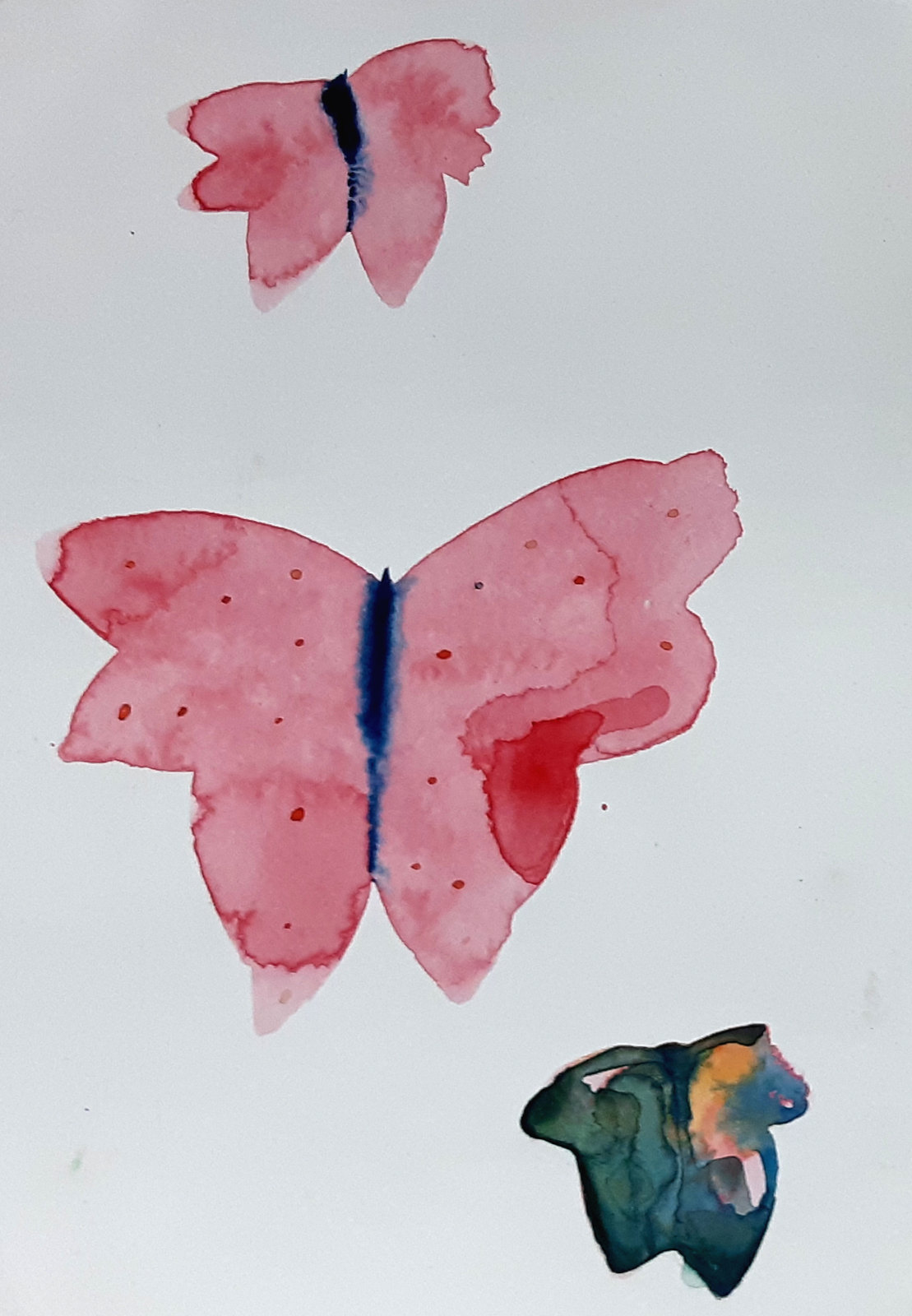This detailed watercolor painting on white paper depicts three distinct butterflies, characterized by their vibrant, blended hues. The top butterfly, small and pink with a dark, almost black-blue center, is delicately rendered. Below it, the largest butterfly showcases a deeper pink tone, adorned with small dots and a dark red spot on the right wing, with a similarly dark blue center. The bottom right butterfly, similar in size to the top one, is predominantly green with hints of yellow on the right and touches of blue. Although the butterflies exhibit a childlike and uneven appearance in their shape and form, the watercolor technique is masterfully applied, achieving a beautiful gradient effect that enhances the overall composition.